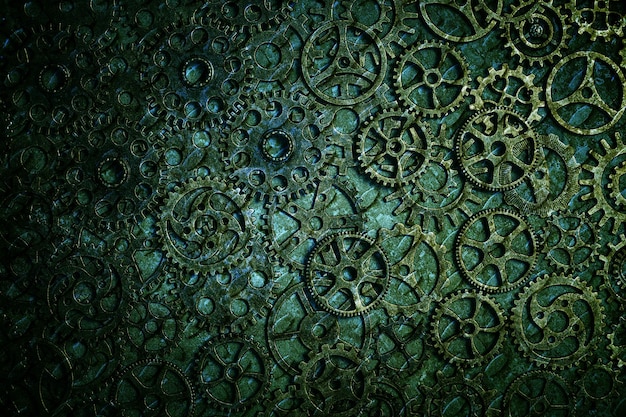This landscape-mode photograph captures an intricate art exhibition piece that evokes a steampunk aesthetic, reminiscent of Jules Verne's 20,000 Leagues Under the Sea. The composition features a myriad of gears—medium-sized and gold-hued—meticulously layered and interlocking with no discernible pattern, creating a dense mosaic of mechanical intricacy. The background transitions from a light green at the center to a much darker, almost black hue at the corners, with the top left and bottom left corners being particularly shadowed, making the gears there barely visible. The top right corner shifts to a bluish tone, providing a better-lit contrast that enhances the visibility of the gears. Centrally, one prominent gear sits above the others, framed against the lighter green, drawing the viewer's eye. The entire piece appears like an exploded view of a clock's inner workings or a complex technological mechanism, potentially functional, adding to its enigmatic allure.